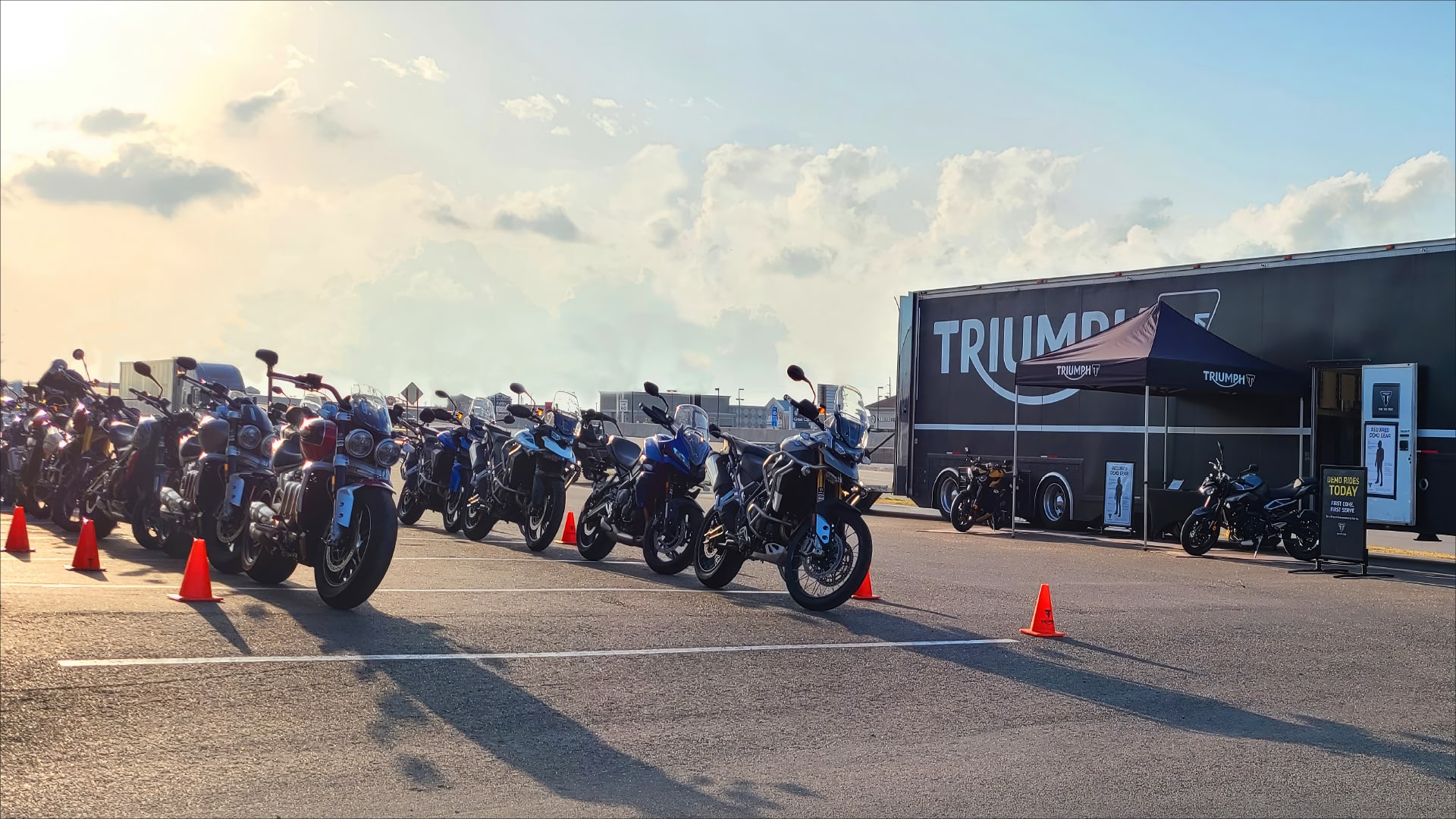This is a horizontal-rectangular photograph of an outdoor motorcycle dealership set in a paved parking lot. Dominating the scene are two rows of motorcycles, all lined up wheel-to-wheel on the gray asphalt, marked by distinct white parking lines running underneath them. Orange traffic cones flank the rows of motorcycles on both sides, enhancing the sense of order. To the right of the motorcycles stands a red-brick building with a white door, bearing the sign "Triumph," indicating the brand of the motorcycles on display.

Adjacent to the brick building is a long black trailer, also emblazoned with the "Triumph" logo in white letters. Next to this trailer, a black pop-up tent is set up, under which a couple of motorcycles are parked, and an entrance to the trailer is visible. The sky above is mostly clear, featuring a blend of low white puffy clouds and a bright spot of sunlight in the upper left, casting a pinkish hue that transitions to a clearer blue towards the right and middle of the image. Notably, there are no people present in the scene, focusing all attention on the neatly arranged motorcycles and the dealership setup.